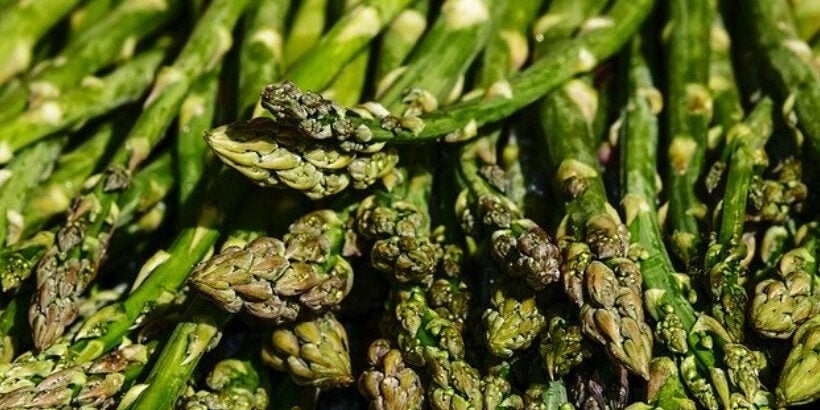This image is an extremely close-up, zoomed-in photo of a stack of asparagus taken outdoors under bright sunlight. The vibrant green stalks dominate the rectangular frame, with their tips and tiny flower buds focused towards the bottom of the image. The asparagus bundles overlap each other, creating small black spaces between the stems. The focus delicately transitions, blurring the stalks as they extend upwards. The image solely features the asparagus, highlighting their texture and natural details without any additional elements or text.